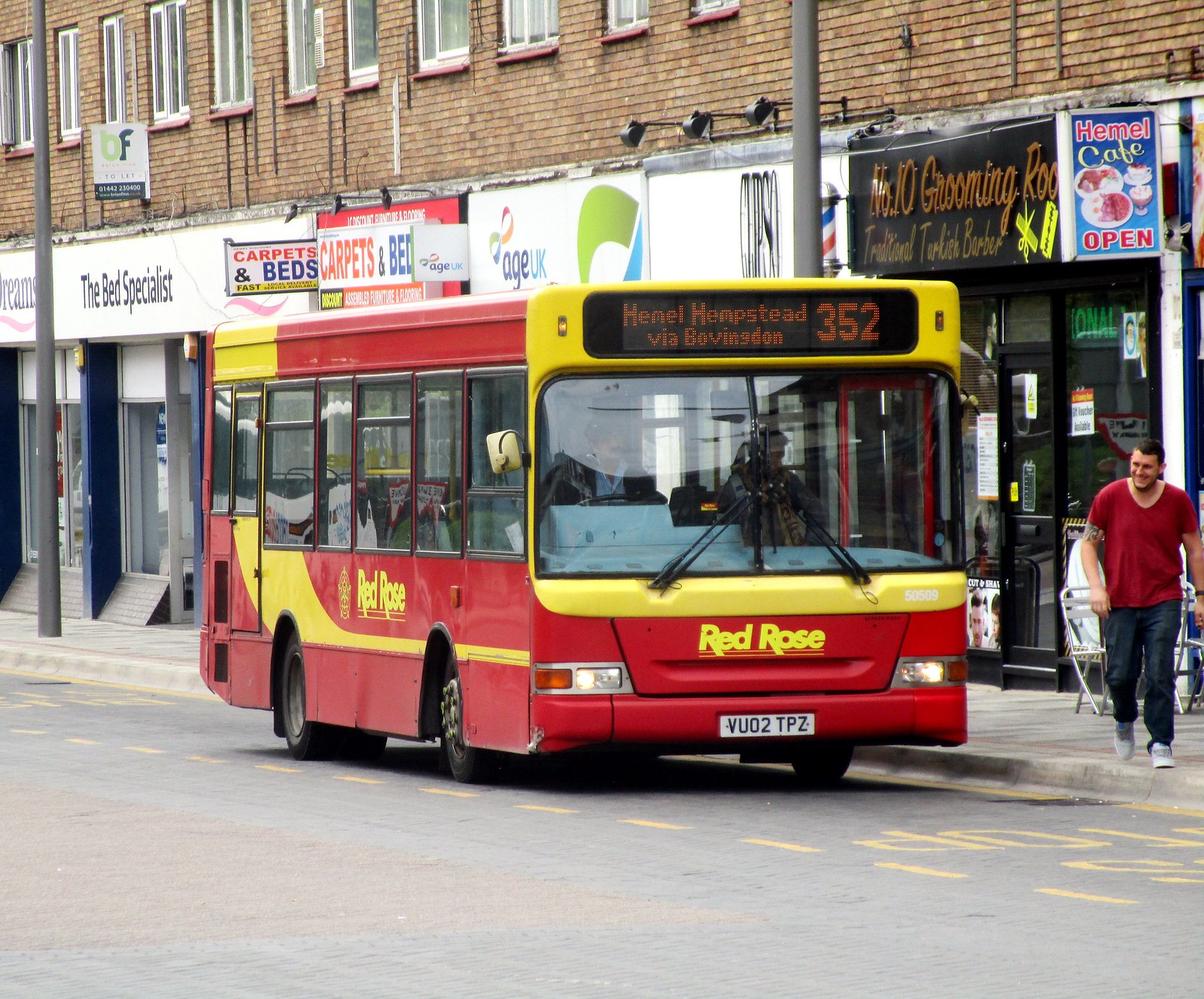The image is a photorealistic scene centered on a large bus driving down a gray-paved city street. The bus is predominantly red with yellow trim and has the words "Red Rose" prominently displayed on the front in yellow lettering. Above the windshield and windows, the destination sign reads "Hemel Hempstead via Bovington" alongside the route number "352." The street features bold yellow writing in the lane the bus is occupying.

Surrounding the bus is a bustling urban environment with bright storefronts, housed in a series of buildings constructed from brown brick. The buildings have multiple windows and host various businesses, such as "Carpets & Beds," "The Bed Specialist," "Dreams," "No. 10 Grooming Room," and "Hemel Cafe," which is noted to be open. 

Towards the right side of the image, a man wearing a red shirt and dark brown pants (mentioned as blue jeans in another description), appears to be walking close to the front of the bus, possibly preparing to cross the street towards the camera.